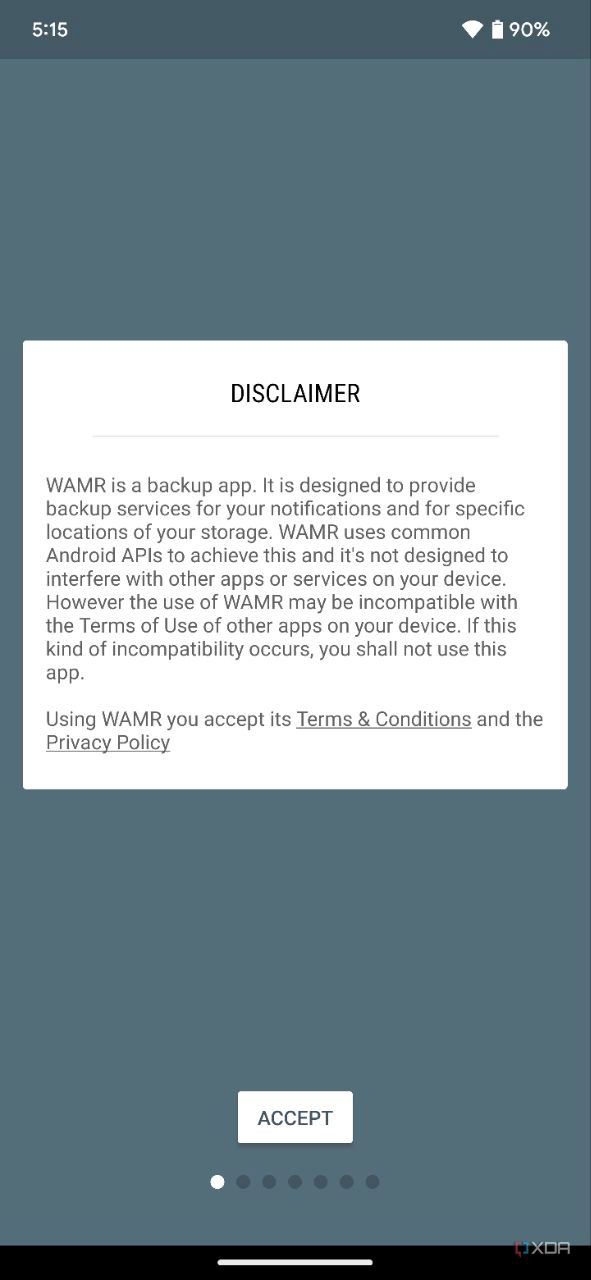This screenshot from a mobile phone displays essential information and a disclaimer within a neatly organized interface. 

- **Top Section**: The top-left corner shows the current time as 5:15, while the top-right corner indicates a battery level of 90% and a cell signal icon. 
- **Background**: The background is a uniform dark grey, providing a stark contrast to the central white box.
- **Central White Box**:
  - **Title**: At the top of the box, "DISCLAIMER" is prominently displayed in uppercase black letters.
  - **Content**: The disclaimer states: *"WAMR is a backup app. It is designed to provide backup services for your notifications and specific locations on your storage. WAMR uses common Android APIs to achieve this and is not designed to interfere with other apps or services on your device. However, the use of WAMR may be incompatible with the terms of use of other apps on your device. If such incompatibility occurs, you should not use this app. By using WAMR, you accept its terms and conditions (underlined) and the privacy policy (underlined)."*
- **Buttons and Navigation**:
  - A white "Accept" button is located at the bottom center of the box.
  - Below this button is a row of six to eight navigation dots, with the first dot highlighted in white, indicating the current page.
- **Watermark**: The bottom-right corner of the screen features a watermark with the text "XDR."

This detailed description captures all the elements presented in the mobile phone screenshot.